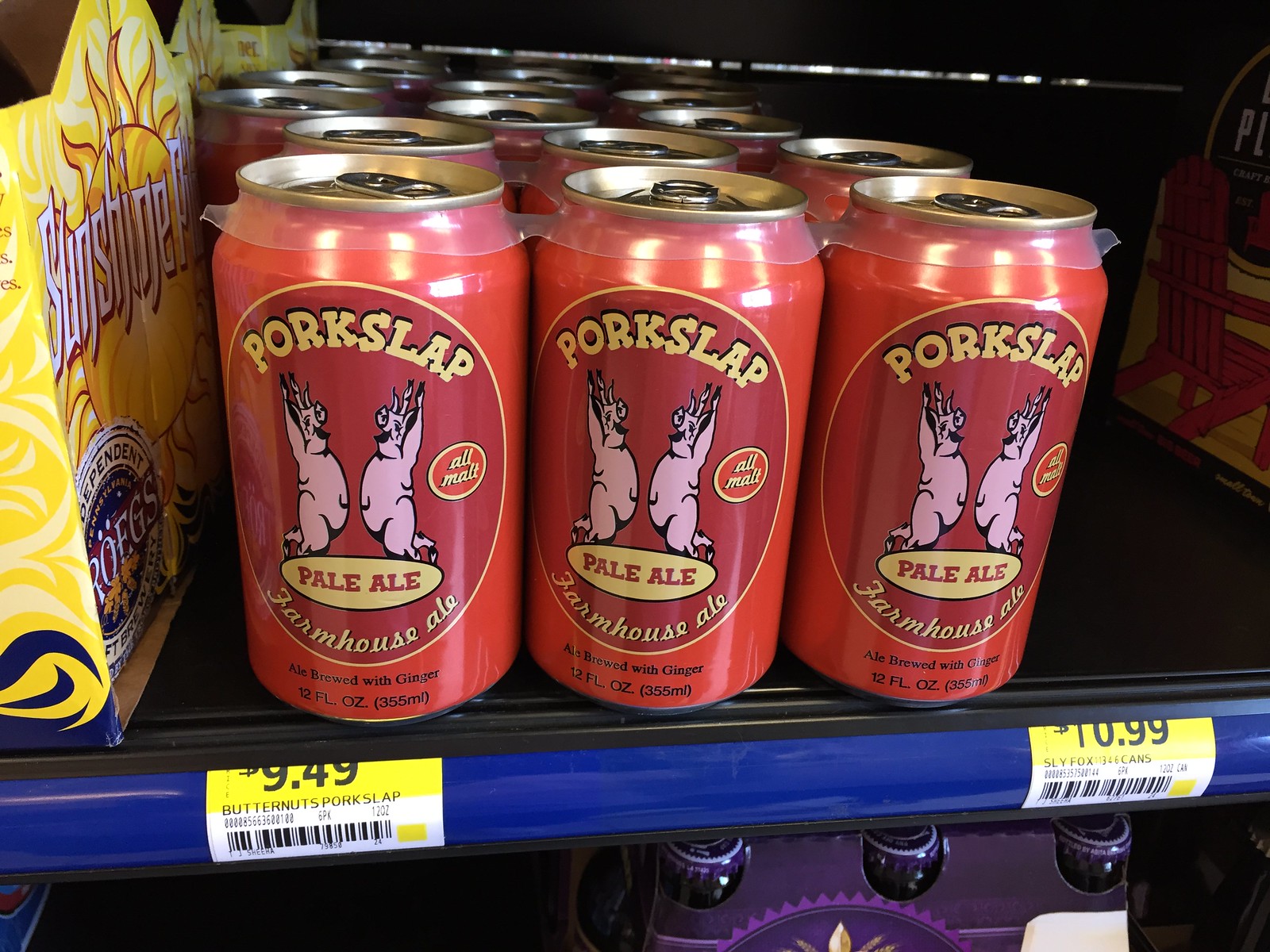This photograph showcases a six-pack of "Pork Slap" pale ale beers on a Walmart shelf, identifiable by the characteristic price tag. The vibrant red cans prominently feature an illustration of two pink pigs with their hands raised upwards. The cans are neatly grouped together in their packaging, which is secured by a standard plastic ring with six slots arranged in two rows of three. Positioned to the left of the "Pork Slap" beers is a yellow cardboard case containing glass bottle beers. Directly beneath this case are three more glass bottle beers held in a purple cardboard container. All beverages are placed on a blue shelf, with the clearly visible bright yellow price tag indicating a cost of $9.49 for the six-pack.